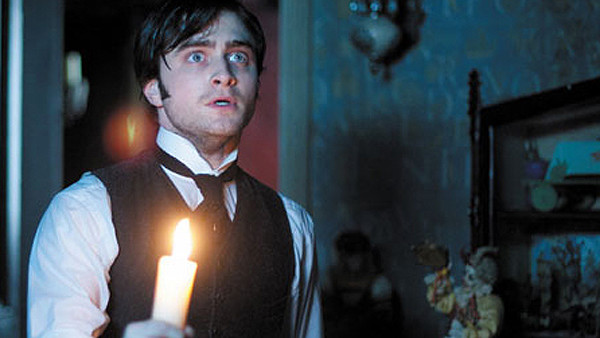This is a detailed screen capture from a still photograph of a movie, featuring the actor Daniel Radcliffe dressed in old-timey attire. He is seen wearing a buttoned black vest and a black tie over a white collared shirt, with the collar folded upward. Radcliffe is holding a single lit candle in his left hand, which casts a warm glow in the dimly lit room. His face, framed by short black hair and dark stubble, shows wide-eyed fear, with his mouth slightly open and nostrils flared. 

The background reveals a richly detailed environment: on the left side, there is a wallpapered wall with a dark brown hutch lined with figurines of clowns, including a doll wearing a red vest with gold arms and a brown hat. The doll's white face holds an object in its left hand. Above Radcliffe's right arm, another clown figurine is partially visible. The scene is further enriched by a blurred yet discernible ceramic ball-shaped light fixture suspended at the top of the photograph. The wall behind Radcliffe is a mixture of gray-beige and red panels, with an open doorway adding depth to the setting. This rectangular photograph captures a moment of suspense and heightened emotion, effectively utilizing both the actor's expressive visage and the intricate background details.